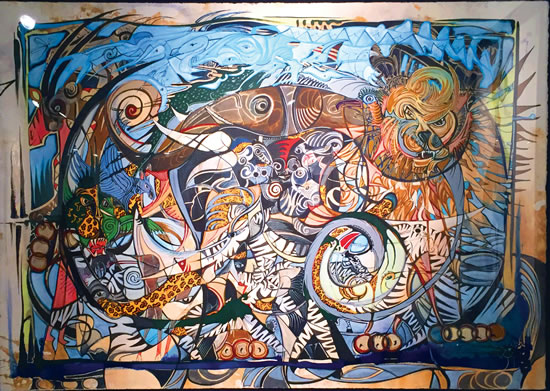This modern, abstract painting, reminiscent of Picasso's style, features a vibrant collage of zoo and African animals. The composition includes fragmented images of elephants, lions, zebras, tigers, giraffes, and possibly a mouse and leopard, intertwined and transitioning into one another, creating a chaotic yet harmonious scene. The painting boasts a rich palette of oranges, blues, browns, reds, and shades of beige, accentuated by geometric features and a stained-glass-like appearance. Scattered elements populate the canvas, avoiding any central focus and enhancing its abstract nature. The top left corner reveals a white dot, possibly a reflection from the photo taken of the actual painting. Framed by a light beige border, this striking piece, with its myriad shapes and decorations, would fit perfectly in an art gallery or museum.